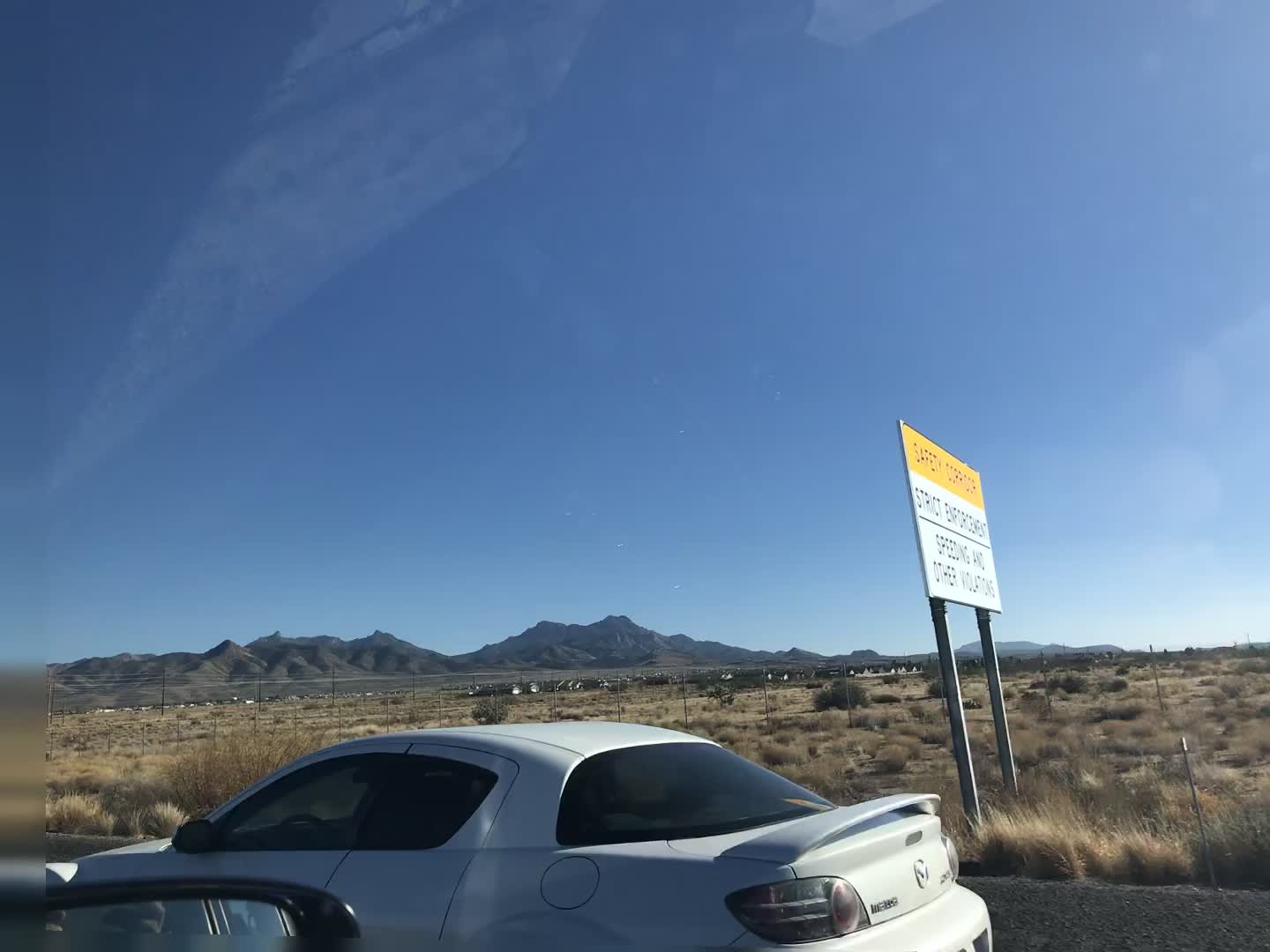A vivid daytime photograph captures the view from the passenger seat of a car, looking out the window. In the lower left corner, the edge of the side view mirror is just visible. The scene unfolds onto a two-lane road, with a white car traveling slightly ahead in the adjacent lane. Beyond the white car, an expansive, arid landscape extends into the distance, characterized by brown earth and scattered patches of scrubby green and brown vegetation. A road sign appears in the frame, though its description is obscured by the angle. Far in the distance, rocky, mountainous hills rise against a backdrop of a mostly clear, blue sky. The overall composition highlights the vastness and rugged beauty of the terrain.